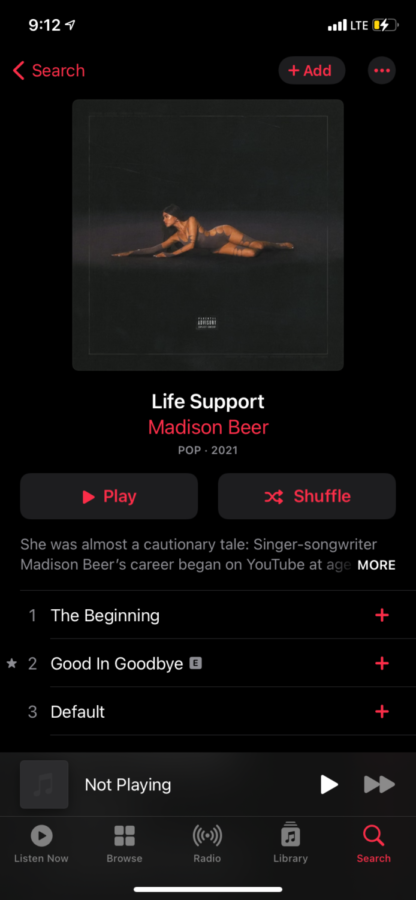Here is a polished and detailed caption for the given image:

---

This screenshot captures the Apple Music app on a cell phone, set against a black background. At the top left of the screen, the word "Search" is displayed in red font, accompanied by a left-pointing arrow icon, indicating a return to the library. On the top right, there is a black bubble icon containing a plus sign and the word "Add" in red font.

Prominently featured below is a large square image of the album cover, centered on the screen. Underneath the album cover, the song title "Life Support" is displayed in bold white letters. Directly below the title, the artist's name is presented in red font. Further down, the genre and the release year of the song are centered and written in white.

Two prominent black buttons are situated beneath this information: the left button is labeled "Play" in red, while the button on the right is labeled "Shuffle." Following these buttons, there is a brief description of the artist, with the word "More" appearing in small white letters on the far right side.

At the bottom of the screen, there is a vertical list of song titles from the album. The first song listed is "The Beginning," with a plus sign displayed to the far right of the title.